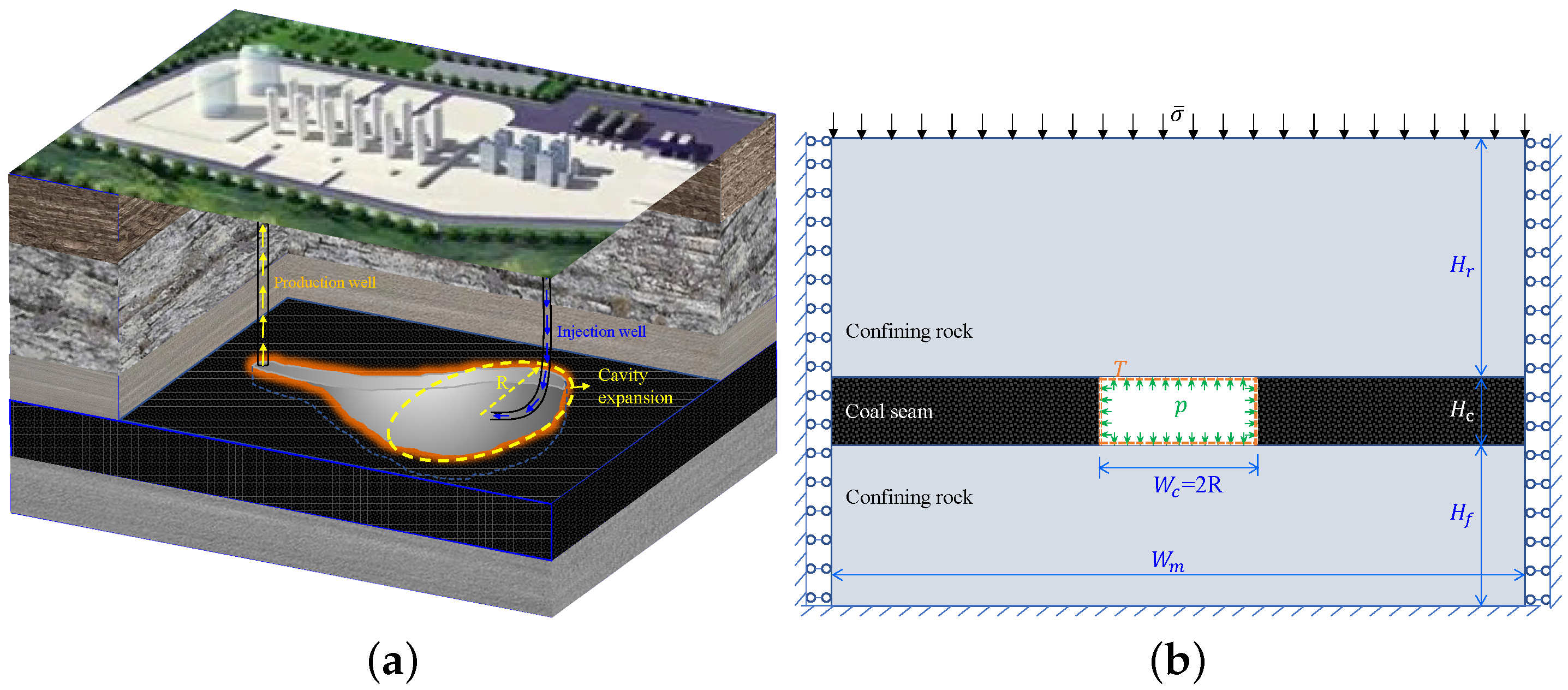The image is a detailed schematic in two parts, labeled (a) and (b), and depicts a mining or fracking operation. Panel (a) on the left shows a cutaway view of the surface and underground structure, featuring a grassy surface with white pavement, container-like buildings, and gray buildings to the right. Below ground, layers of brown and gray rock lead to a silver pool connected by two tubes, with dashed yellow and red lines measuring a cavity expansion. Blue arrows indicate an injection well on the right, while yellow arrows denote a production well on the left, illustrating the extraction process. The surface appears to blend a satellite photo with a computer-simulated underground.

Panel (b) on the right presents a simplified side view, colored light blue, with black arrows at the top and blue circles on each side. It includes a black bar with a white rectangle and mathematical symbols, labeled "confining rock" and "coal seam" in black letters, with additional details like green pressure arrows and a dashed red line marked with the letter T, denoting the pressures within the coal seam.